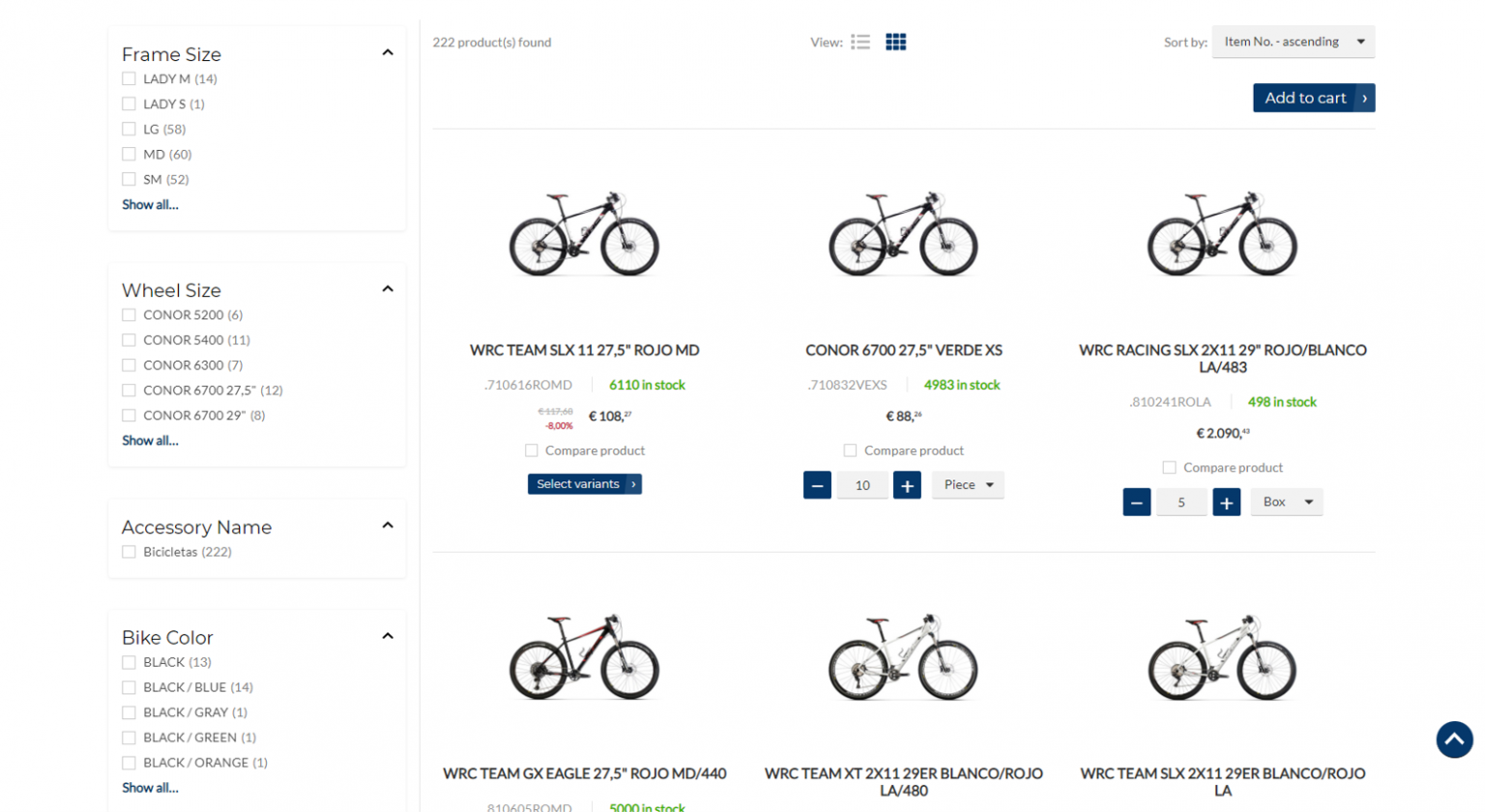The image depicts a detailed interface of an online shop specializing in bicycles and related accessories. 

**Left Side: Filtering Options**
The left sidebar is dedicated to a variety of filtering options to help users narrow down their product search. 
- **Frame Size**: Options include ladies M, ladies S, F, G, M, D, S, M. A blue "Show All" button can be clicked to expand the list.
- **Wheel Size**: Choices are presented from smallest to largest, including 500, 600, and 700.
- **Accessory Name**: Users have a "PC Select" option.
- **Bike Color**: Available colors are black, black and blue, black and gray, black and green, and black and orange.

**Right Side: Product Listings**
The right section showcases the search results with details pertaining to 222 products found. Users can select their preferred view between a list format and a grid format, with the grid format currently active. The products are sorted by item number in ascending order.

Each product entry has specific details:
1. **WRC Team SLX**:
   - Stock: 6,110 available
   - Price: 108 euros
   - Buttons: A green "In Stock" indicator and a blue "Select Variant" button.

2. **Kona 6700 Vette SX**:
   - Stock: 4,983 available
   - Price: 8.26 euros
   - Feature: Text box for entering the desired quantity

3. **WRC Racing Blanco**:
   - Stock: 4,988 available
   - Price: 2,090.43 euros

4. **WRC Team GX Eagle**
5. **WRC Blanco Orojo**
6. **Blanco Orojo LA**

Highlighted prominently within each product entry is the stock availability and pricing, ensuring customers have clear visibility for making purchase decisions. A notable blue "Add to Cart" button is centrally positioned for easy access.